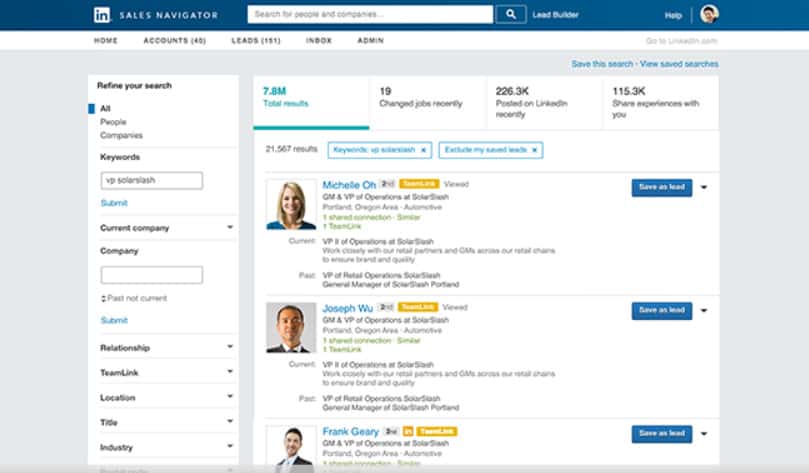At the top of the interface, there is a long blue bar featuring a white square with the letters "IN" inside. To the right of this, the phrase "Sales Navigator" is displayed. Below the blue bar is a search bar with the placeholder text "Search for people and companies" alongside an image of a magnifying glass.

Directly below the search bar, an indication of "7.8 million total results" is underlined in blue. Additional stats include "19 changed jobs recently," "226.3K posted on LinkedIn recently," and "115.3K share experiences with you."

The content then showcases three individuals:

1. **Michelle O**: 
   - **Profile Picture**: A woman with short blonde hair, smiling.
   - **Title**: QM and VP of Operations.
   - **Action**: A blue rectangle with "Save as Lead."

2. **Joseph Wu**:
   - **Profile Picture**: A man probably in his late 40s, sporting a neutral expression.
   - **Title**: VP of Operations.
   - **Action**: A blue "Save as Lead" rectangle.

3. **Frank Geary**:
   - **Profile Picture**: A man likely in his late 20s, dressed in a suit.
   - **Title**: VP of Operations.
   - **Action**: A blue "Save as Lead" rectangle.

Each of these entries includes a profile image, name, job title, and the option to "Save as Lead" in a prominent blue box on the right.